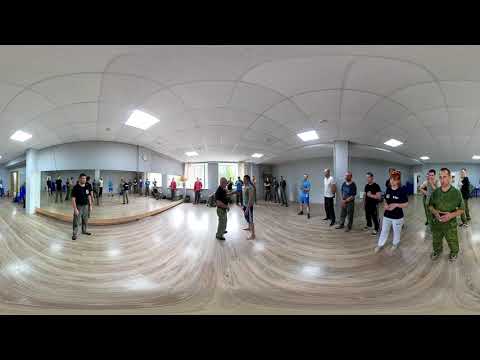In this panoramic, fisheye lens photo capturing an expansive indoor space, the scene unfolds within a large room featuring a wooden floor and a billowed tile ceiling adorned with numerous lights. Dominating the center of the image, two men are engaged in what appears to be a serious conversation, with one man touching the shoulder of the other. This interaction draws the attention of a predominantly male audience, many of whom are dressed in military or police uniforms, hinting at a possible teaching program or military-related event.

The composition includes several groups of people: to the right, individuals form a line, while on the left, others stand on a raised platform. Notably, these groups stand beneath lights fixed to the ceiling, emphasizing the room's structured lighting arrangement. The background showcases two large picture windows, with natural daylight streaming in, indicating it's likely midday. A man dressed in red stands in front of these windows, adding to the room's dynamic.

Despite the panoramic view, it’s clear there are no chairs, and people are casually dressed, some in short pants. The raised platform or stage also lacks seating, reinforcing the sense that this is a standing-only event. The visual depth is accentuated by poles on both sides of the room, and a door is visible on the left, providing an additional point of interest. The overall ambiance is one of focused engagement amidst a spacious, well-lit indoor setting.